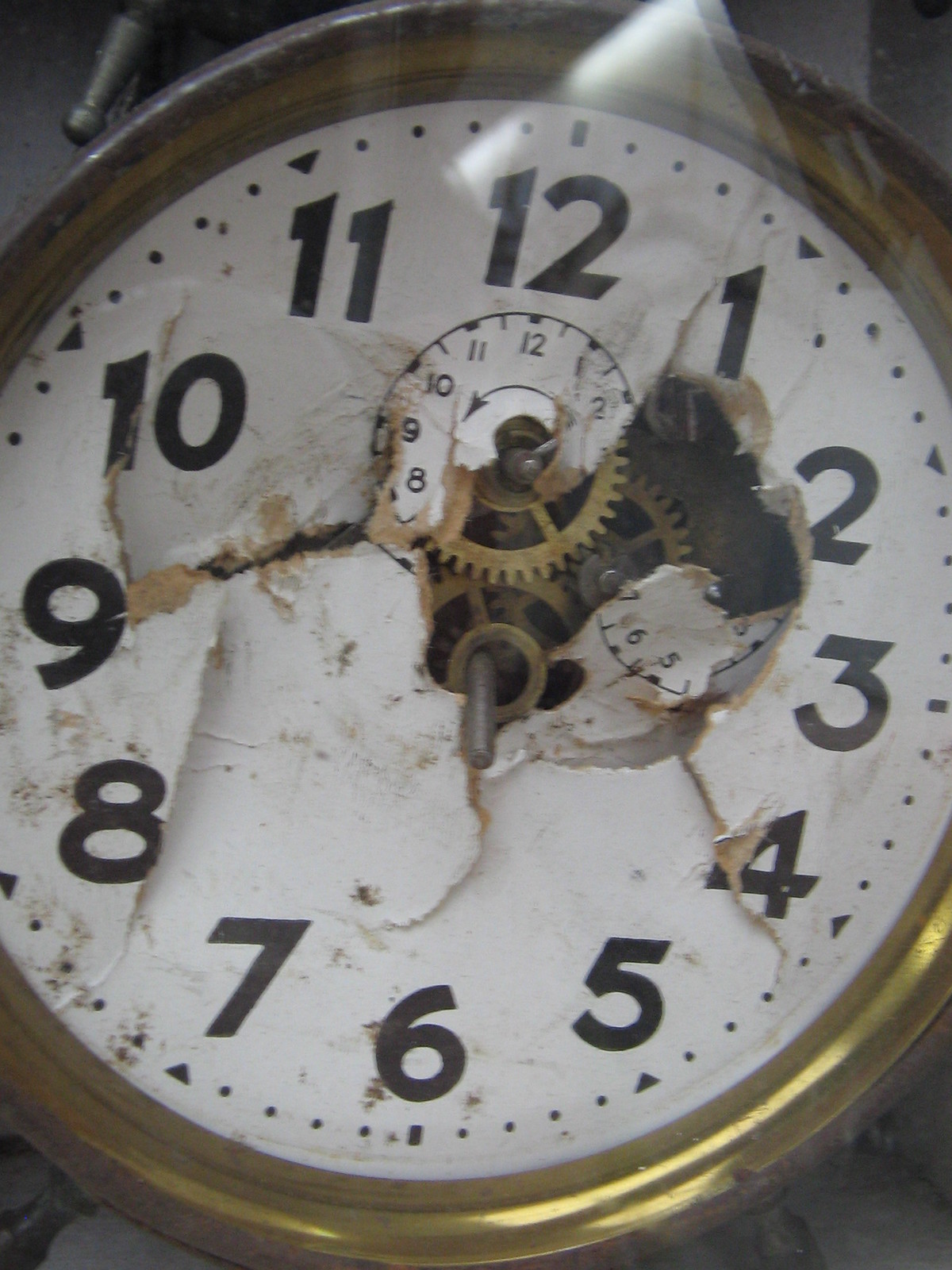In this image, we see an old, broken clock with a transparent covering made of either plastic or glass. The clock's interior is significantly damaged. Its white center, which appears to be made of particle board or cardboard, features black block numbers arranged in a clockwise fashion from 1 to 12. Notably, the clock is missing its hour, minute, and second hands, leaving a hole in the middle that provides a clear view of its inner workings. Inside, we observe intricately designed gears, likely made from copper or a gold-like material. The clock also has a decorative border that appears to be brass or gold.